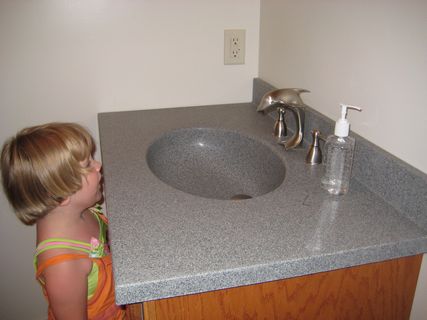In this color photograph, a small girl stands inside a bathroom sink, her nose nearly level with the countertop, illustrating her petite stature. She has short, blonde hair with bangs that just touch her forehead. The countertop is a solid surface resembling faux gray granite, accompanied by an integrated sink. The vanity base is made of oak-colored wood, complementing the sleek countertop.

The girl is dressed in a sleeveless lime green shirt paired with an orange sleeveless dress. She gazes intently at the faucet, which is whimsically designed to resemble a dolphin, complete with a spout that appears to emulate the dolphin's mouth. The faucet comprises a uniquely mounted setup: the left and right handles are separately installed, requiring three distinct holes.

Beside the faucet is a clear pump bottle with a white top, likely containing hand sanitizer given the clear liquid inside. An ivory-colored electrical outlet is visible on the white back wall, reinforcing the sterile and sparse ambiance of the bathroom, which may be recently built or remodeled as suggested by the lack of additional furnishings or decoration.